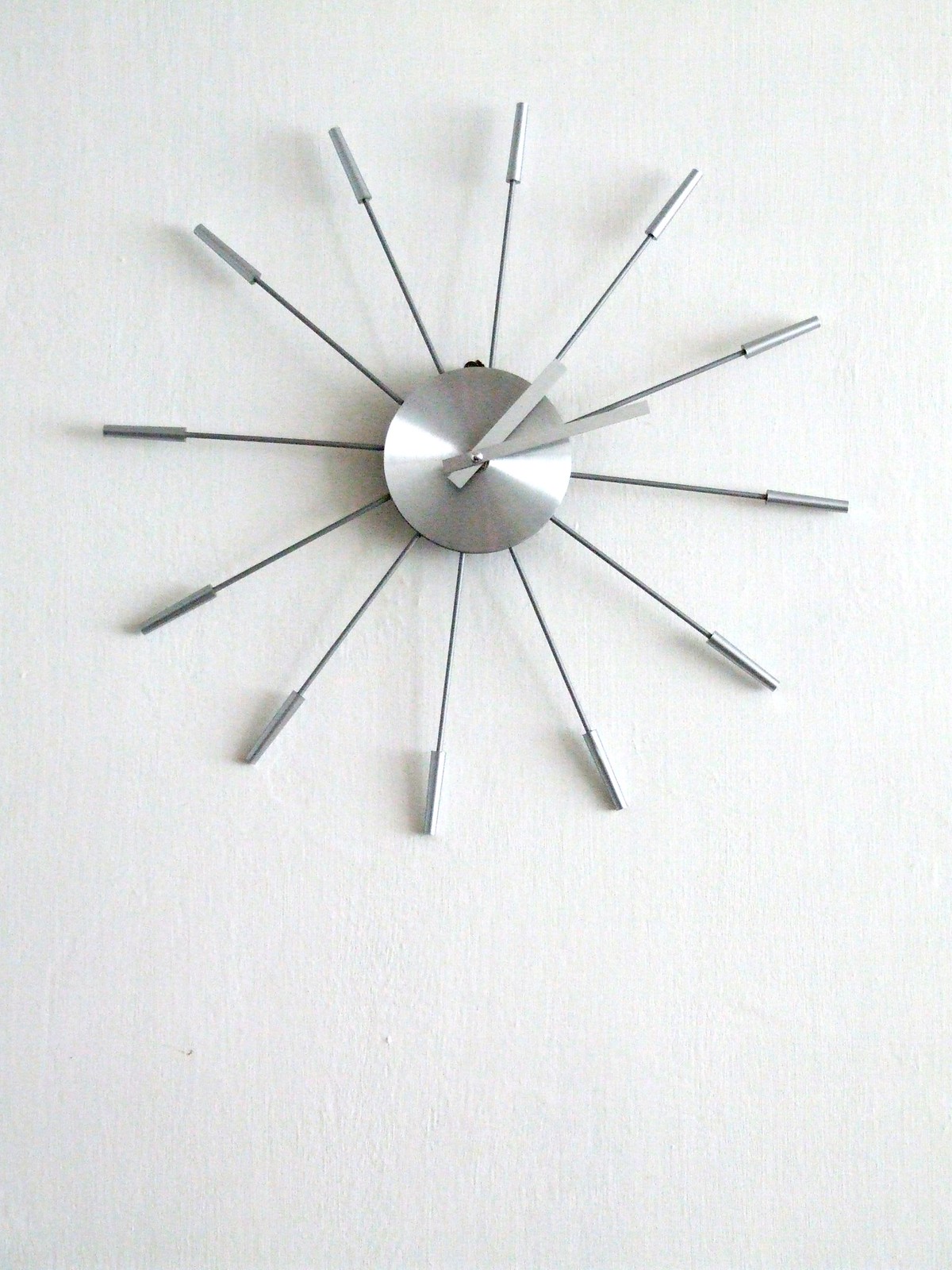The image showcases a unique wall-mounted clock against a textured cream-colored wall, which features subtle brush strokes giving it an intentional design. The clock is distinctively minimalist, comprising a central small metallic circle housing a rivet that joins two gray hands—an hour hand and a minute hand. The face of the clock lacks traditional numbers. Instead, 12 slender white rods radiate outwards like spokes of a star, each capped with small metallic tubes, representing the hour markers. The clock appears slightly askew, with the hour hand positioned just past the one marker and the minute hand slightly beyond the second marker, indicating a time of 1:11. Fine lines on the clock's white background and the subtle imperfect alignment add a touch of modern artistic flair.